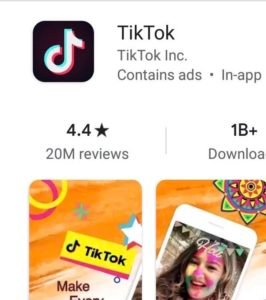This image is a detailed screenshot snippet of the TikTok app's download page in the app store. At the very top, a thin, light gray horizontal line runs across the screen. Positioned in the upper left corner is the TikTok app icon, which appears as a black, rounded-square containing the TikTok musical note symbol. This symbol is predominantly white with light blue accents and a reddish shadow to its right. Adjacent to the app icon is the brand name "TikTok" in bold black text. Directly beneath it is the gray subtext "TikTok Inc.", followed by another line indicating "Ads · In-App Purchases".

Further down, the app's ratings and review details are displayed. It shows a 4.4-star rating based on 20 million reviews. Next to this, separated by a vertical dividing line, is the download count, partially obscured but indicating over 1 billion downloads (not fully visible as it cuts off after the "A" in "Downloads").

At the bottom of the screenshot, two different phone outline screenshots are visible against an orange background. The first image features a yellow box displaying the TikTok music symbol and the "TikTok" name. In the center, the text begins with "Make" but the rest is not visible. This area is decorated with colorful, TikTok-themed symbols like rings and stars. The second image shows part of a cellphone screen with the image of a young female, complemented by an artistic, modern chic sketch of a multi-point star in green, blue, yellow, and red hues.